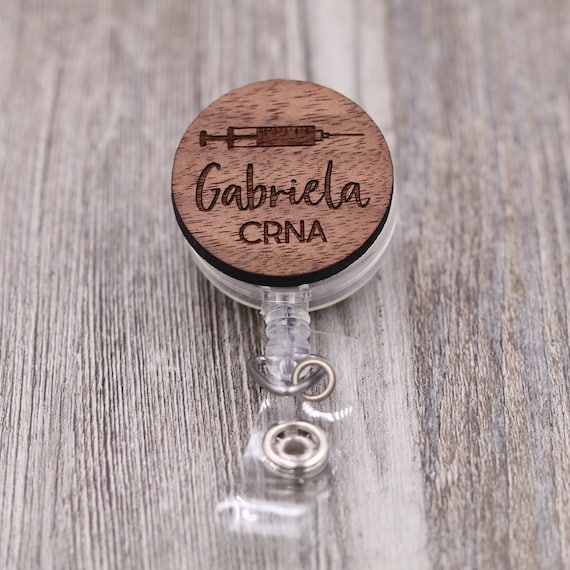In the photograph, a wood table with varying shades of gray, brown, and off-white provides the background. Resting on the table is a unique piece of jewelry. The base of the jewelry consists of a circular silver piece, from which a triangular silver element extends. Hanging from this triangular element is another small silver circle. Additionally, a white plastic component is integrated into the design.

At the forefront, a small circular wooden disc, in a pale chocolate brown color, lies atop the jewelry, bearing detailed chocolate brown graphics. The graphics depict a syringe, which is approximately three-quarters full and includes a needle at its tip. Below the syringe illustration, the text "Gabriella, C-R-N-A" is inscribed in matching chocolate brown font.